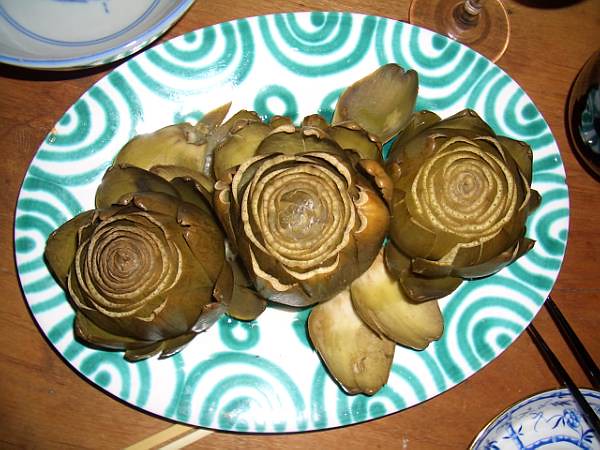The photograph captures a detailed overhead view of a culinary presentation featuring three artichoke hearts, meticulously arranged on an oval-shaped, white paper plate adorned with green spiral and arch patterns along the edges. The artichoke hearts, resembling rose flowers, display a gradient of dark green outer petals transitioning to lighter green centers, some petals are tucked under. The plate is placed on a light brown wooden table. Additional elements in the scene include a portion of a porcelain plate with two chopsticks on the lower right, part of a white porcelain bowl with a blue rim on the upper left, and the base of a champagne glass near the top right, completing the intricate table setting.